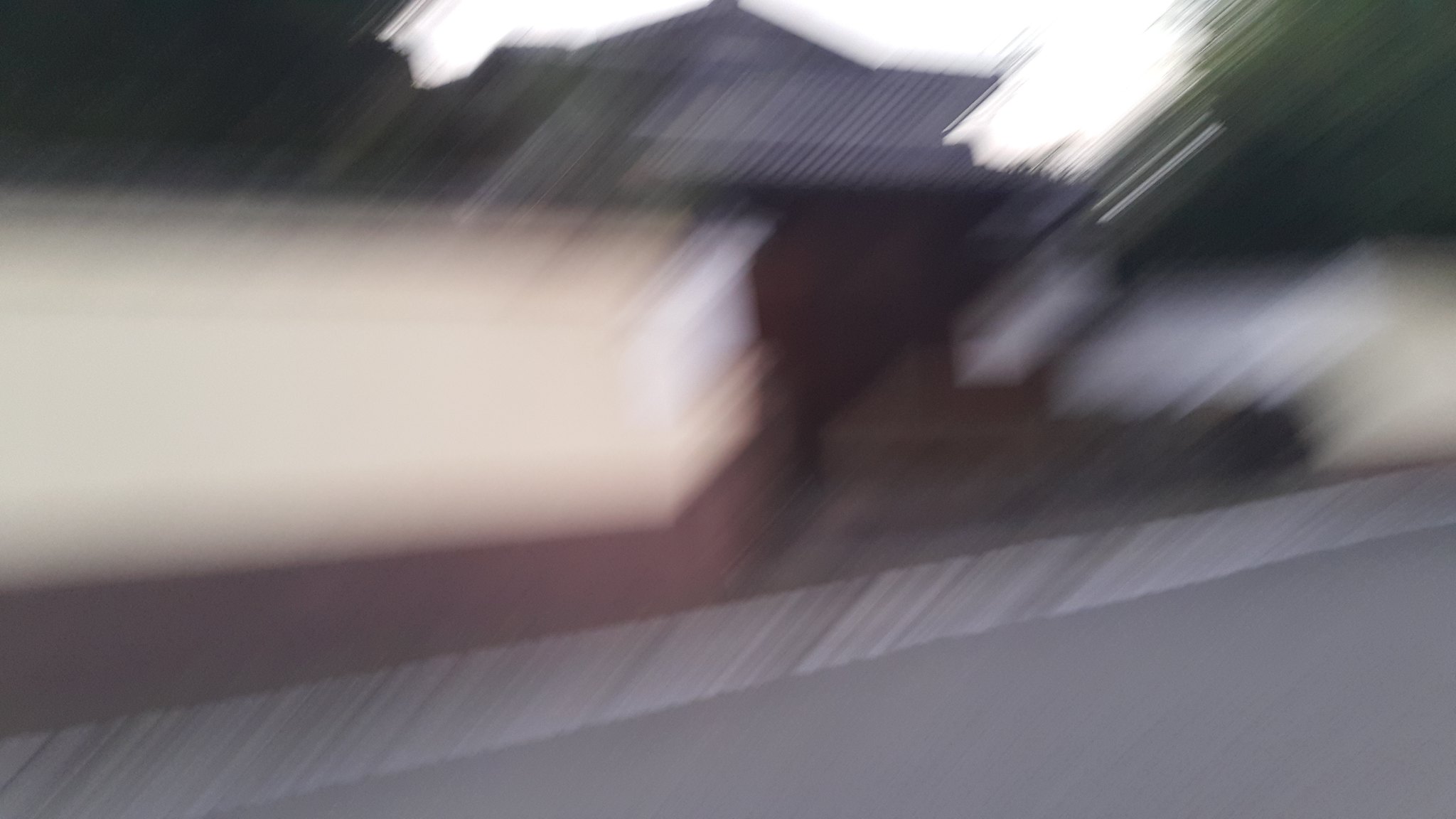The photograph is extremely blurred, likely taken from a vehicle moving at high speed. At first glance, the image shows what appears to be the front of a house set in an outdoor environment. The building features a white peaked roof, and below it is a mixture of gray, darker gray, lighter gray, and brown patches, suggestive of different materials or lighting effects. Bordering the house, there's a red brick fence with a white wooden top, flanked by a curb and pavement of slate gray. Surrounding the blurred, undefined structure, the sky transitions from white to light blue, and dense, green trees frame the scene on either side. The upper corners of the image display a stark contrast, appearing very dark, possibly indicating more trees or shadows. Despite the lack of clarity, the combined elements suggest a red brick house in a lush, tree-lined area.